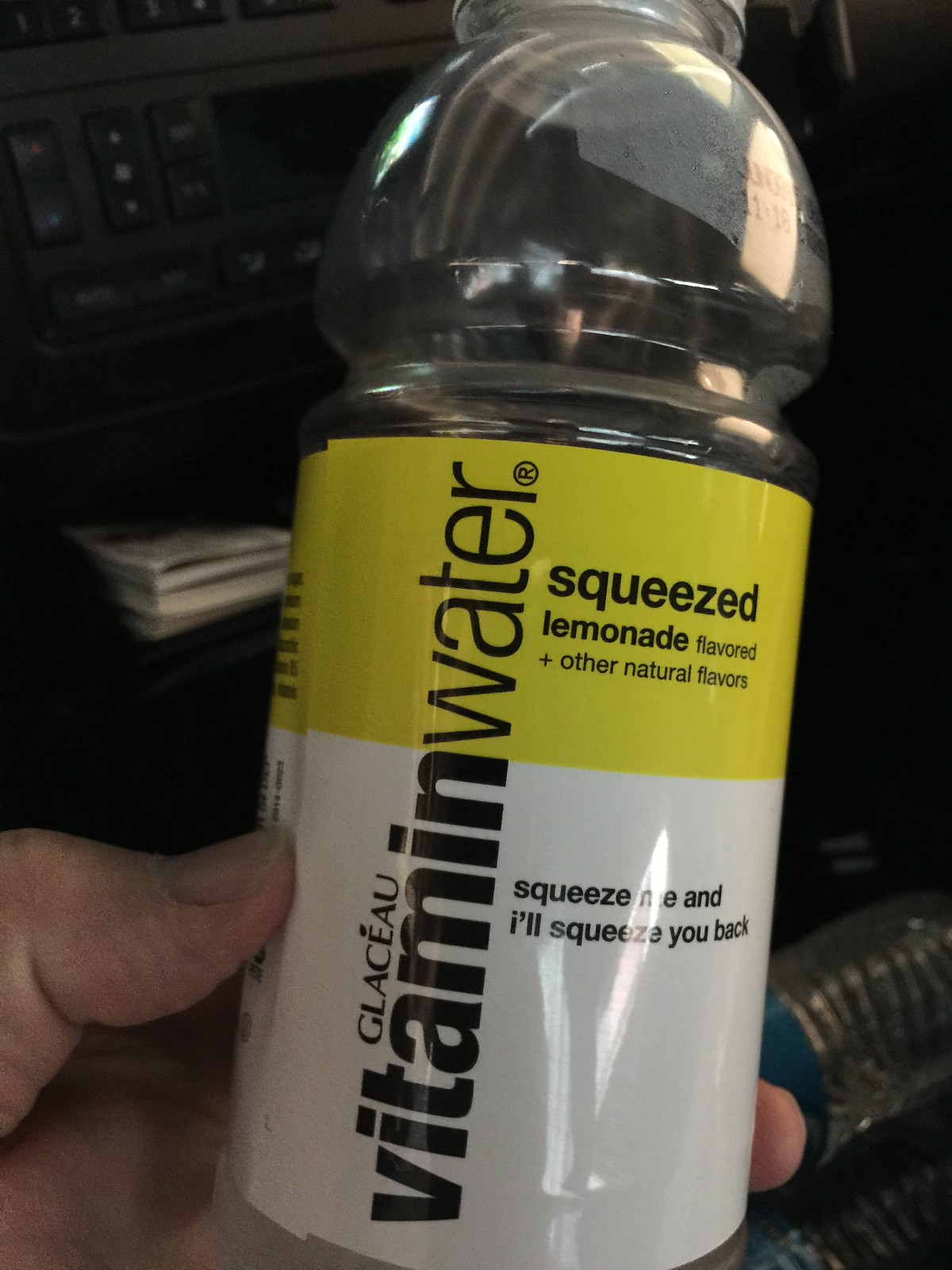The image depicts a slightly vertical shot of a male Caucasian hand holding a small bottle of Glaceau Vitamin Water. The bottle is crafted from clear plastic and features a distinctive label split into two color segments: a vibrant yellow occupying the top third and an immaculate white covering the bottom two-thirds. Dominating the label, the brand name "vitamin water" is inscribed vertically from bottom to top. The brand "GLACEAU" is printed perpendicular to the main label text. Within the yellow section, the flavor is clearly stated as "Squeezed Lemonade, Flavored and Other Natural Flavors." Below, in the white section, the quirky message "Squeeze one and I’ll squeeze you back" is visible. The grip only partially reveals the thumb and the first couple of fingers, which are positioned towards the bottom of the slightly tilted container. This scene is set against a predominantly dark, almost black, background, which draws attention to the bottle and the details on its label.